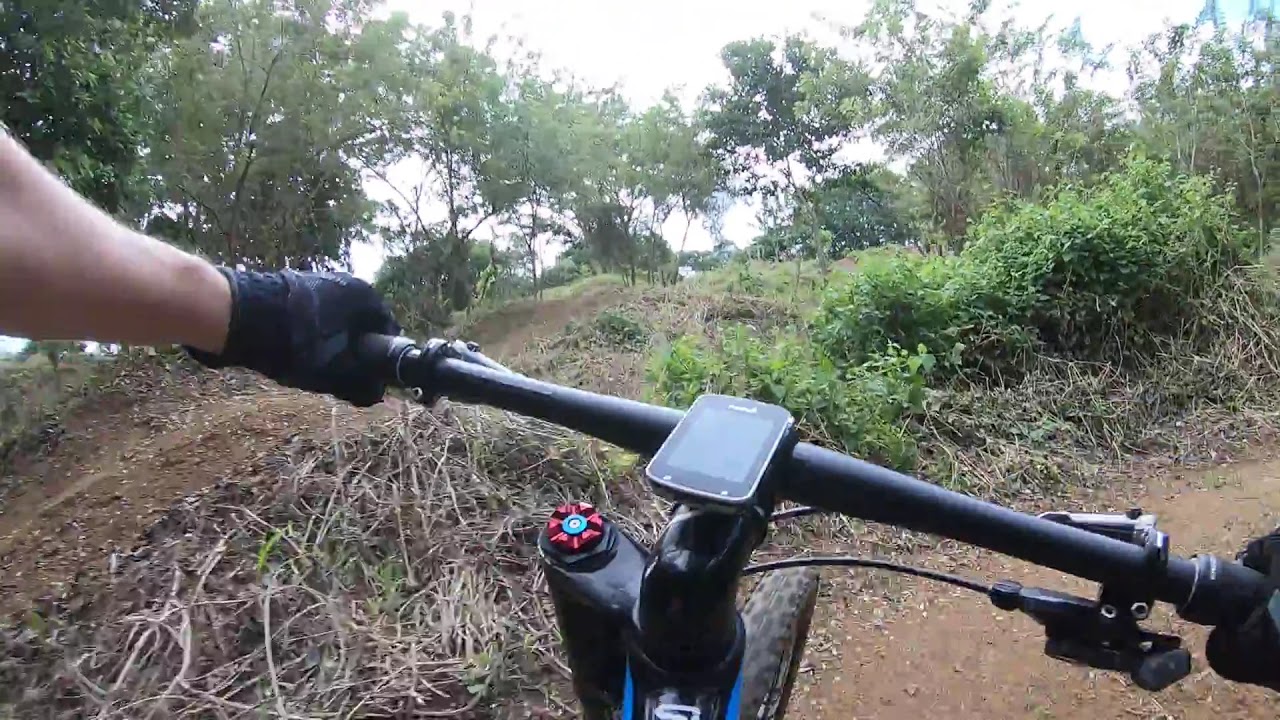In this detailed image, we see a person riding a mountain bike along a dirt nature trail from a first-person perspective, likely captured with an action camera mounted on their chest. The handlebars are black, with a cell phone securely placed in a center holder. The rider's hands, clad in black gloves, grip the handlebars tightly as they navigate the twisting path. In the foreground, the bike's knobby front tire makes contact with the brown dirt trail, lined with a mix of shrubbery, reeds, and green-leaved bushes. A mounted water bottle can be seen on the fork of the bike. The upper portion of the image reveals a tree-dotted landscape with a white, overcast sky peeking through the branches, suggesting a blend of overgrowth and bare ground perfect for mountain biking. To the left, a wavy dirt hill rises, indicative of a trail feature designed for jumps and other mountain biking activities.